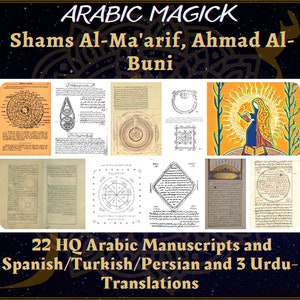This image appears to be an advertisement or information graphic for a book related to Arabic magic, specifically titled "Arabic Magic," spelled with a 'K' as "MAGICK." The book is seemingly called "Shams al-Ma'arif," authored by Ahmad Al-Buni. The advertisement is set against a black background and prominently features various shades of white and off-white text detailing the content.

At the top, the text prominently displays "Arabic MAGICK." Below this title, there is further text: "Shams Al-Ma'arif Ahmad Al-Buni." The central part of the image showcases several rows of pages from the book. In total, 22 high-quality Arabic manuscripts are highlighted, available in Spanish, Turkish, Persian, and also in three Urdu translations.

A closer look at the central pages reveals detailed graphics and diverse styles of writing. The first page is orange, adorned with a circular graphic. The second page is white with a conical drawing and other intricate graphical writings. The third page boasts a cream-colored, aged appearance with writing at the top left and a prominent spiral graphic at the center bottom.

To the left, there is a white page featuring a circle at the top and a square at the bottom. Adjacent to this, a vibrant illustration on an orange background captures a woman with long blonde hair reading a book, flanked by green vines and set against a sunlit backdrop. She is garbed in a blue and red robe. Below these primary images, more pages are displayed featuring an array of squares, circles, spirals, and text in varying hues of white and off-white, though the details are less discernible.

This detailed composition effectively showcases the rich and varied manuscripts included in this collection, making it a captivating and informative representation of "Arabic MAGICK."